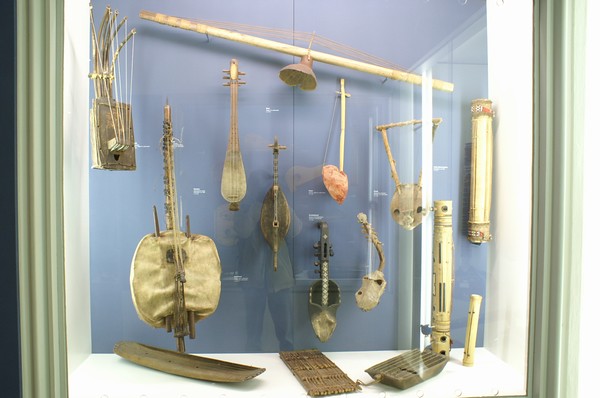The photograph captures a display of several unique and antique musical instruments, primarily string instruments, arranged against a long wall. The collection appears to be from various cultures and eras, showcasing the diversity and historical significance of these pieces. At the top left, a square, box-shaped acoustic guitar can be seen, followed by an intriguingly-shaped instrument with keys on its side, resembling a vacuum bag. The top right features a long, slender instrument that could be an elongated cello or violin. On the far right, there are more unusual and colorful instruments, with hints of pink and white. Below, there are smaller, raft-like objects, including a rectangular brown piece and a light green one. The scene appears to be viewed through a window with a white frame, possibly in a museum or exhibition, with some objects displayed on a white platform table and others hanging from metal bars. A light fixture is also suspended among the instruments, adding to the eclectic mix of the display.